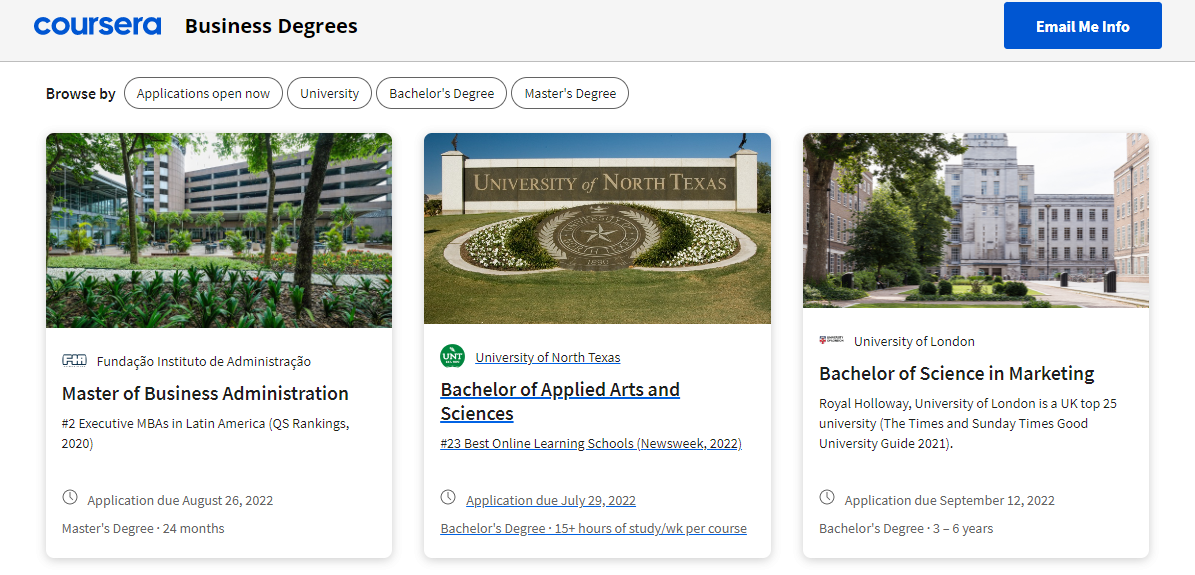The image features a clean, white background with a large blue box at the top. Inside this box, "Coursera" is prominently displayed in blue text, accompanied by "Business Degrees" in black text. Directly below, there's a blue button that reads "Email me info."

On the right side, there is a navigation option labeled "Browse by," which includes circled categories: "Applications Open Now," "University," "Bachelor's Degree," and "Master's Degree."

Below this section, there are three detailed boxes with images and information about various degree programs:

1. The first box showcases an image outlined in blue, depicting a university. The program title "Master of Business Administration" is displayed, with a small blue box in the corner indicating the application deadline as August 26, 2022. It also mentions that the degree is a master's program, typically completed in 24 months. This program is offered by a university with a picture included.

2. The second box contains an image of the University of North Texas. It features a green circle with the university’s name and the program title "Bachelor of Applied Arts and Sciences." It specifies the application deadline as July 29, 2022, and notes that this bachelor's degree requires 15+ hours of study per week per course.

3. The third box displays an image of a large university, identified as the University of London. It offers a "Bachelor of Science in Marketing," with the application deadline set for September 12, 2022. This bachelor’s degree program can take between three to six years to complete.

Each section is richly detailed, emphasizing application deadlines, duration, and study requirements for prospective students interested in pursuing business degrees.